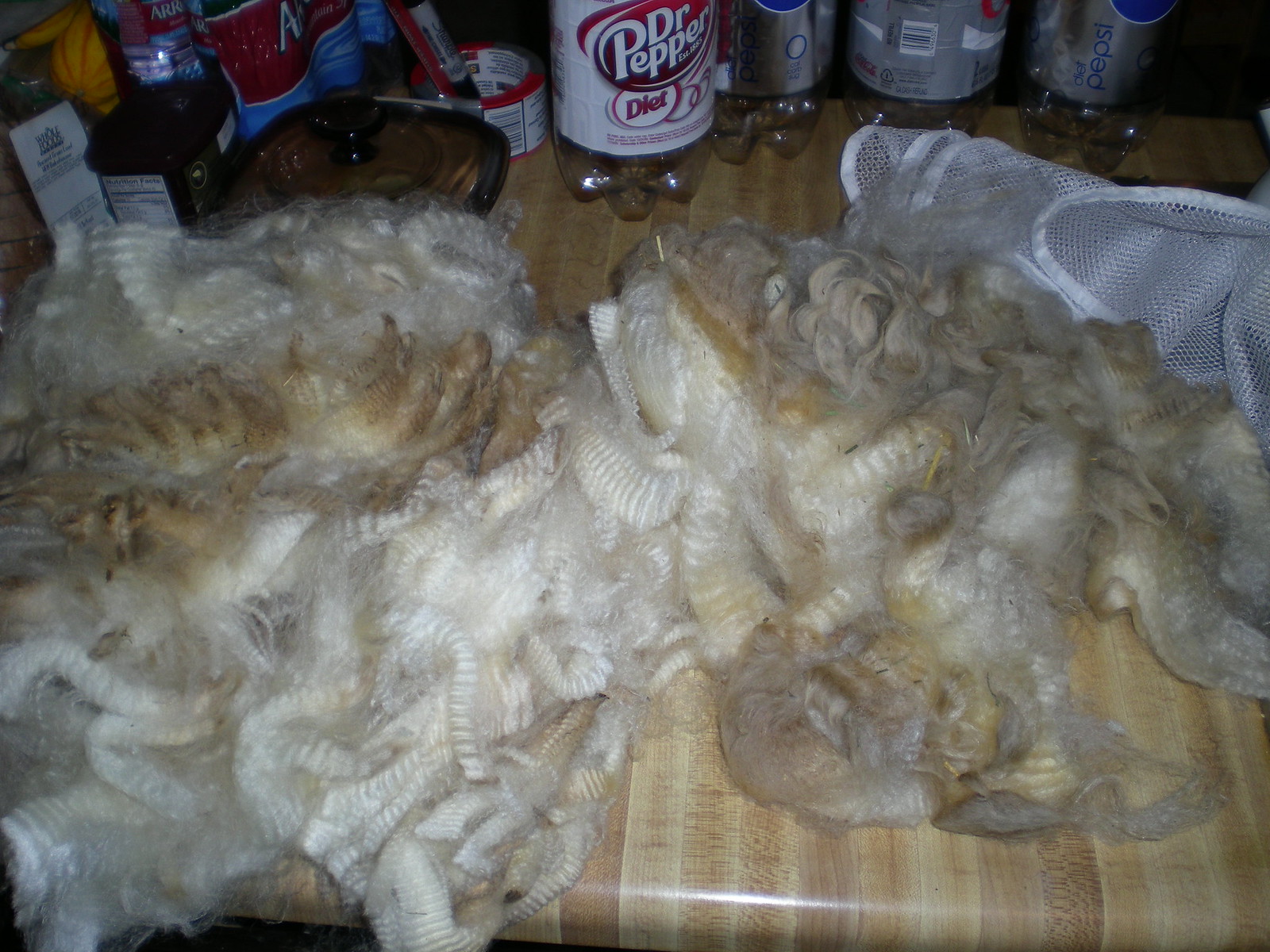This photograph depicts a cluttered brown, cheap-veneered wood table or countertop, likely situated in someone's home or apartment. The table is strewn with an assortment of peculiar and ambiguous items, primarily dominated by a spread of fur that appears organic, yet possibly faux, marked with white, brown, and gray shades. The fur, reminiscent of a stuffed animal's texture, lies amidst a background populated with various empty beverage bottles including a Diet Pepsi, a Dr. Pepper, and several clear bottles with white and gray labels. Additionally, there's a green bottle with a white label and a red and blue bottle. In the upper left corner, one can spot a glass lid and a roll of tape, while a piece of white netting is visible to the right. These elements collectively create an enigmatic and eclectic scene.